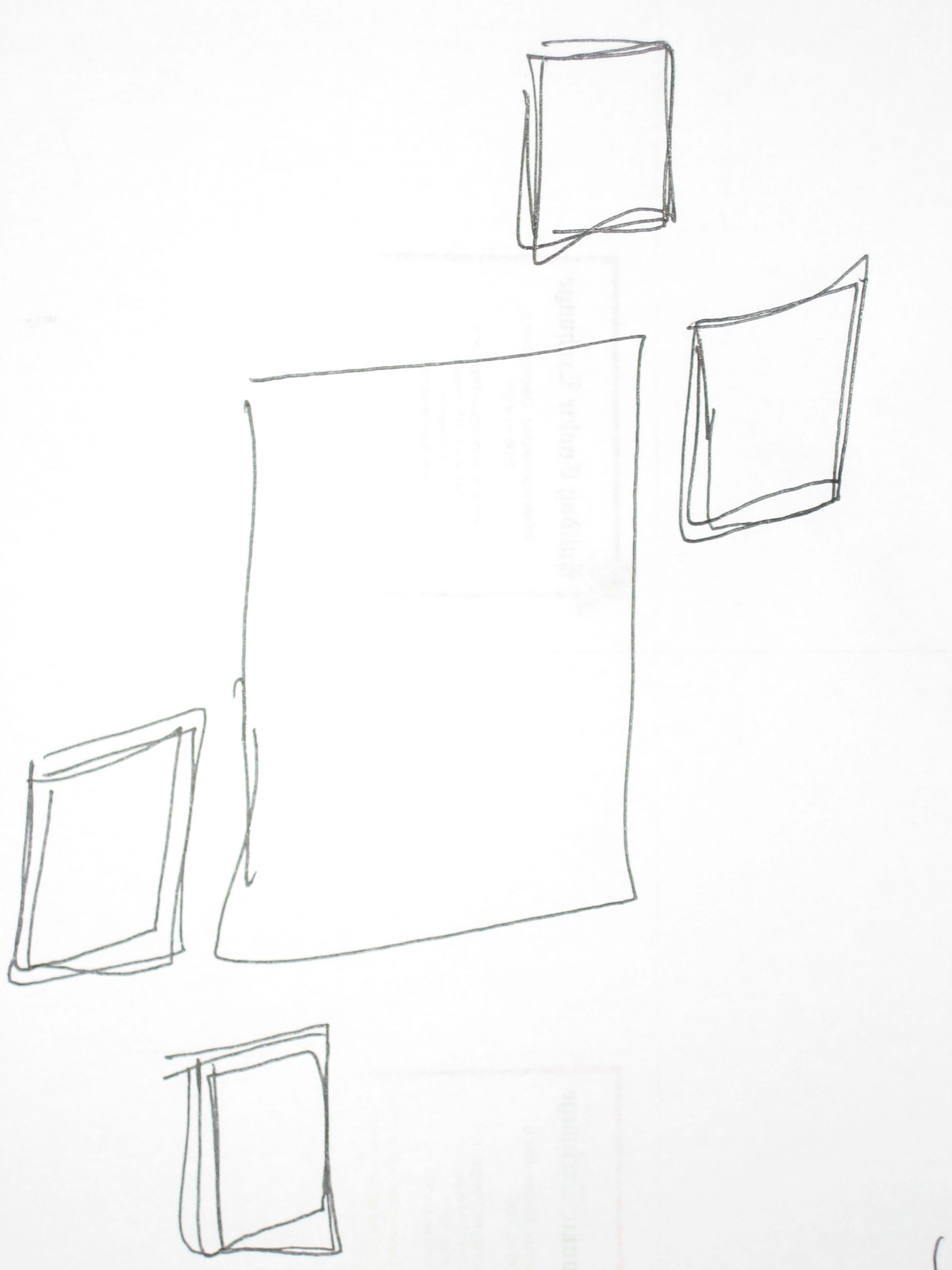This image is a detailed pencil drawing set on a piece of white, portrait-oriented paper, likely of letter size. The composition features four distinctive squares and one rectangle, all of which have been hand-sketched with varying degrees of outline reinforcement.

In the upper right section of the paper, though not completely in the corner, there is a square that has been outlined several times, giving it a dense, textured appearance. Directly below it and slightly to the right is another square, similarly outlined multiple times. 

To the left of the second square, a large rectangle is sketched with a single, clean line, contrasting with the heavily outlined squares surrounding it. Horizontally aligning with the base of the rectangle and residing towards the bottom edge of the paper, not completely reaching the corner, is the third square, also reinforced with multiple outlines. 

Finally, towards the bottom left of the paper, aligning with the bottom of the rectangle, is the fourth square, diagonally opposite to the top-right square. These squares form an implied diagonal line running from the upper right to the lower left edge and from the top-right square to the bottom-left square.

The overall arrangement of these geometric shapes, with their varying intensities of outline and their strategic positioning, creates a visually engaging and intricate abstract composition.